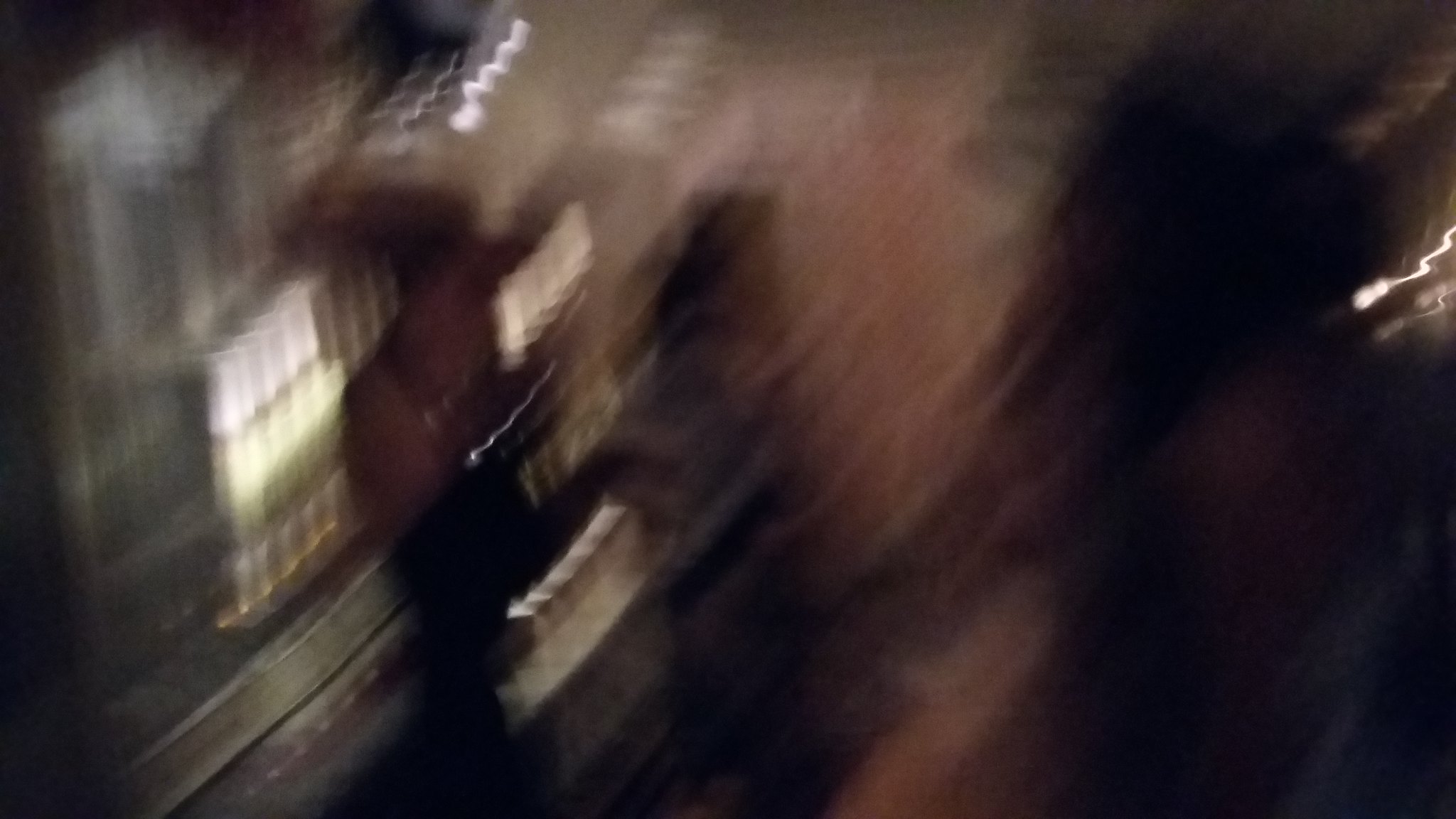The image is a highly out-of-focus, blurry photograph that appears to depict three women. On the right side of the image, a woman with long, brown hair is visible, standing at an angle with her left shoulder facing towards the left side of the photo. She is wearing a strapless, sleeveless dress made of white fabric, noticeable despite the blur. To the left, there is a blonde woman adorned with silver bracelets which appear as silver streaks on her arm. Her hair is styled in an updo, creating an effect that makes the hair look stretched out behind her, almost as if she is in motion. A third woman is discernible in the center background, though she appears as a mere blur with indistinct brown hair.